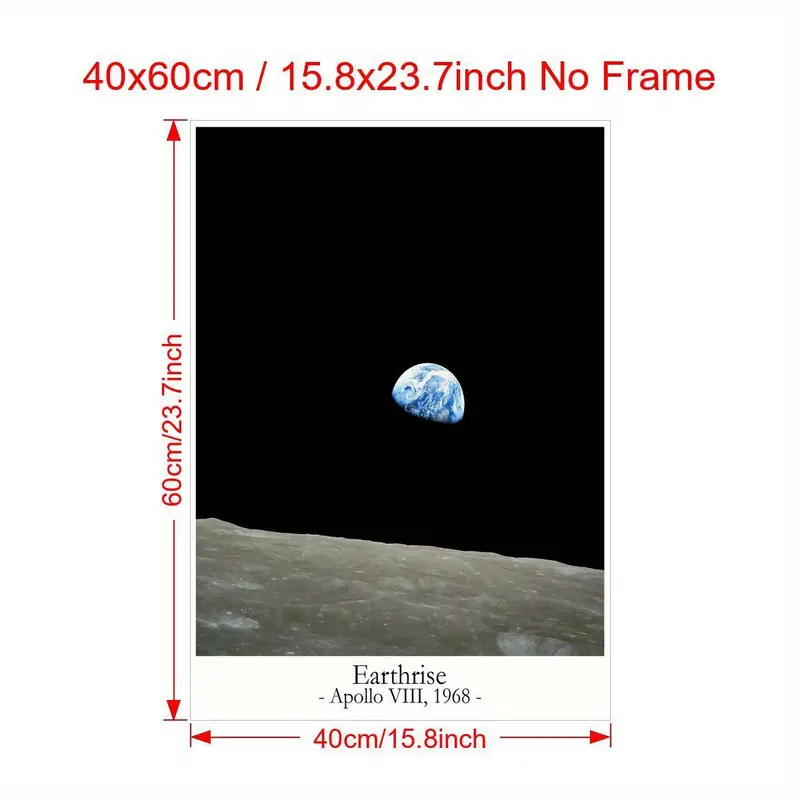This striking photograph, titled "Earthrise, Apollo 8, 1968," captures a unique perspective of the Earth as seen from the Moon's surface during the historic Apollo 8 mission. The Earth appears as a half-illuminated blue and white marble with splotches of brown, reminiscent of a lunar phase, set against the inky blackness of space. A gray, white-speckled portion of the Moon's surface is visible at the bottom of the image, providing a stark contrast to the vivid planet above.

The photograph also contains specific measurements and labels, likely indicating its suitability for a poster. At the top and bottom of the image are red arrows with dimensions: 40 x 60 centimeters (15.8 x 23.7 inches), and additional measurements along the sides, confirming the size of the poster. This detailed information, presented with arrows, seems to enhance the scientific and commercial appeal of the image, inviting viewers to appreciate both its artistic and historical significance.